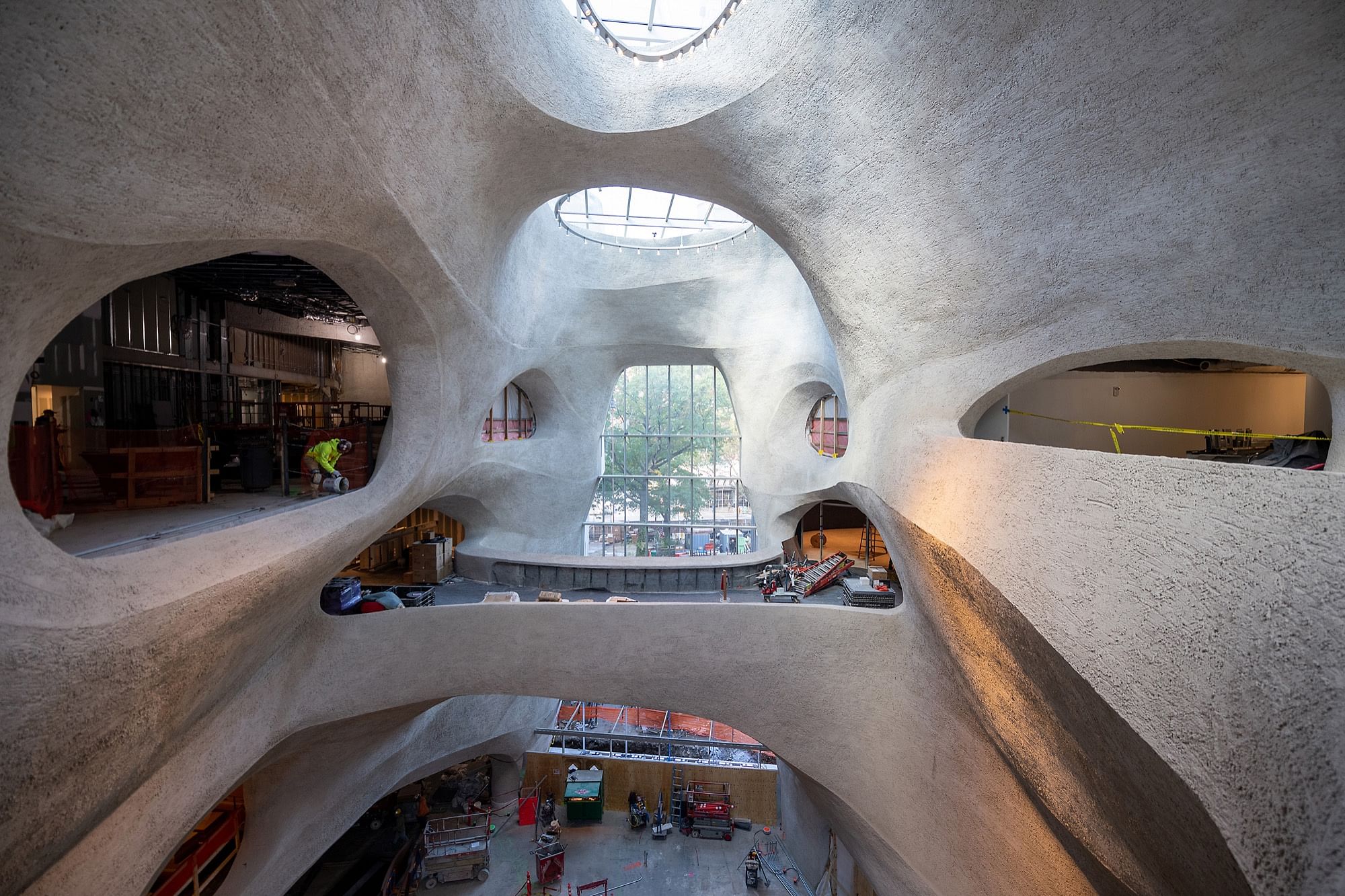The image depicts the interior of an extraordinary, curvilinear building resembling the whimsical style of architect Antoni Gaudí. The structure appears to be either a fantastical museum or a futuristic residence, possibly even an AI-generated scene or a highly stylized photograph. The walls and windows follow organic, naturally shaped contours, giving the impression of rooms carved out of a giant stone or resembling a cave. Sunlight spills into the space through numerous skylights and large windows, illuminating the intricate details.

From our vantage point on an upper floor, we see multiple levels below, where construction appears to be ongoing. Workers in bright yellow jackets and t-shirts are visible, as well as construction materials, bare floors, ladders, and small platforms. Wooden furniture is arranged in one of the rooms to the left, adding a touch of warmth to the stone-like environment. An overpass-type bridge connects sections of the upper levels, creating a dynamic, interconnected layout.

Additional details include a central window below the skylight and what seems to be a balcony or ledge in the middle section. A person in a bright yellow jacket is seen leaning down to the left, while yellow caution tape lines one of the curved exhibit walls on the right, reinforcing the notion that this may be a museum still in the process of setting up its exhibits.